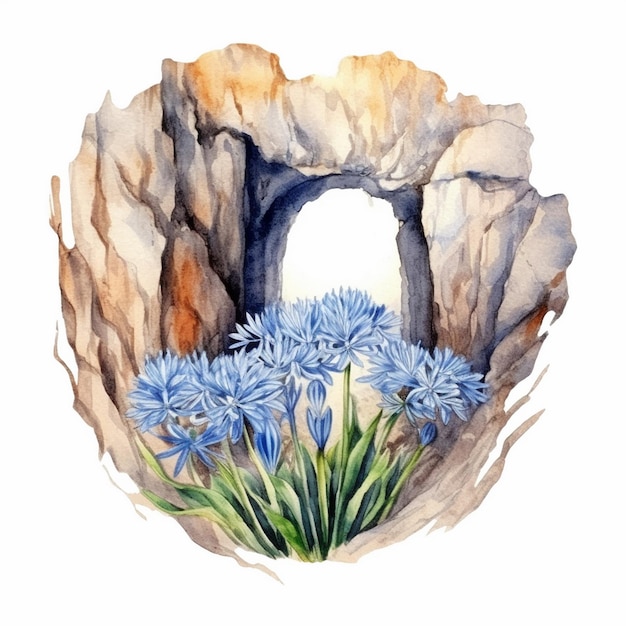This watercolor painting vividly captures a scene where vibrant blue flowers, with their dainty and elegant petals, bloom from rich green stems. The flowers, detailed with some buds yet to open, stand gracefully at the forefront of the image. These flowers are set against a beautifully textured rock formation that resembles a stone archway or cave. The rock surface displays a variety of earthy tones, from beige with gentle hints of yellow, to sections tinged with rust and brown hues. The archway creates a captivating focal point with its heart-like shape and an opening that leads into a white passage, enhanced by the bright, white background behind the entire scene. This art piece skillfully blends the natural elegance of the flowers with the rugged, yet warm, textures of the stone formation.